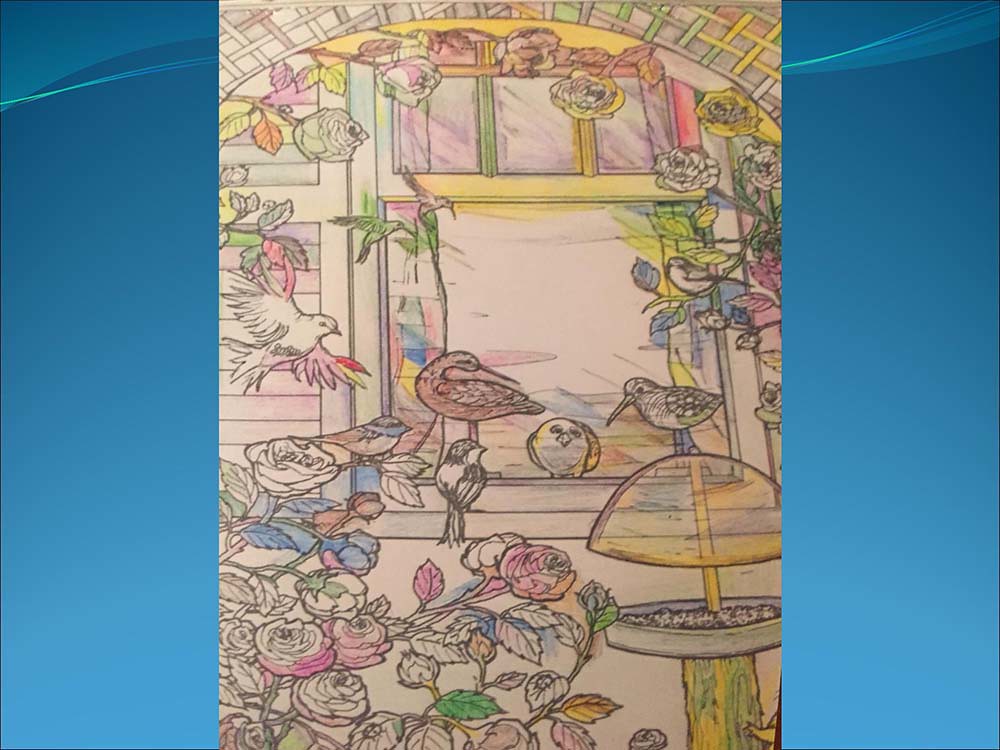This vibrant illustration, reminiscent of a meticulously colored page from a coloring book, is rendered with colored pencils and sits atop a flat blue surface, possibly a screen or desktop background. The scene features an enchanting bird feeder adorned with a roof, positioned in the bottom right corner, and flanked by an array of intricately detailed birds of various species—distinguished by their diverse beak shapes, both long and short. A scene of lush flora comprises the left side, where elegant rose bushes flourish, their vines cascading overhead to form a picturesque canopy above a quaint window. The backdrop is a striking mix of light yellow, green, pink, purple, and blue hues, set against a soft pinkish-white background that mimics the texture of paper. The terrace, enhanced by an intricate patterned arch at the top of the drawing, adds architectural beauty and depth to the scene. Overall, the colors and composition create a serene, almost magical ambiance, expertly highlighted in dark gray outlines that delineate the fine details of the coloring book style.